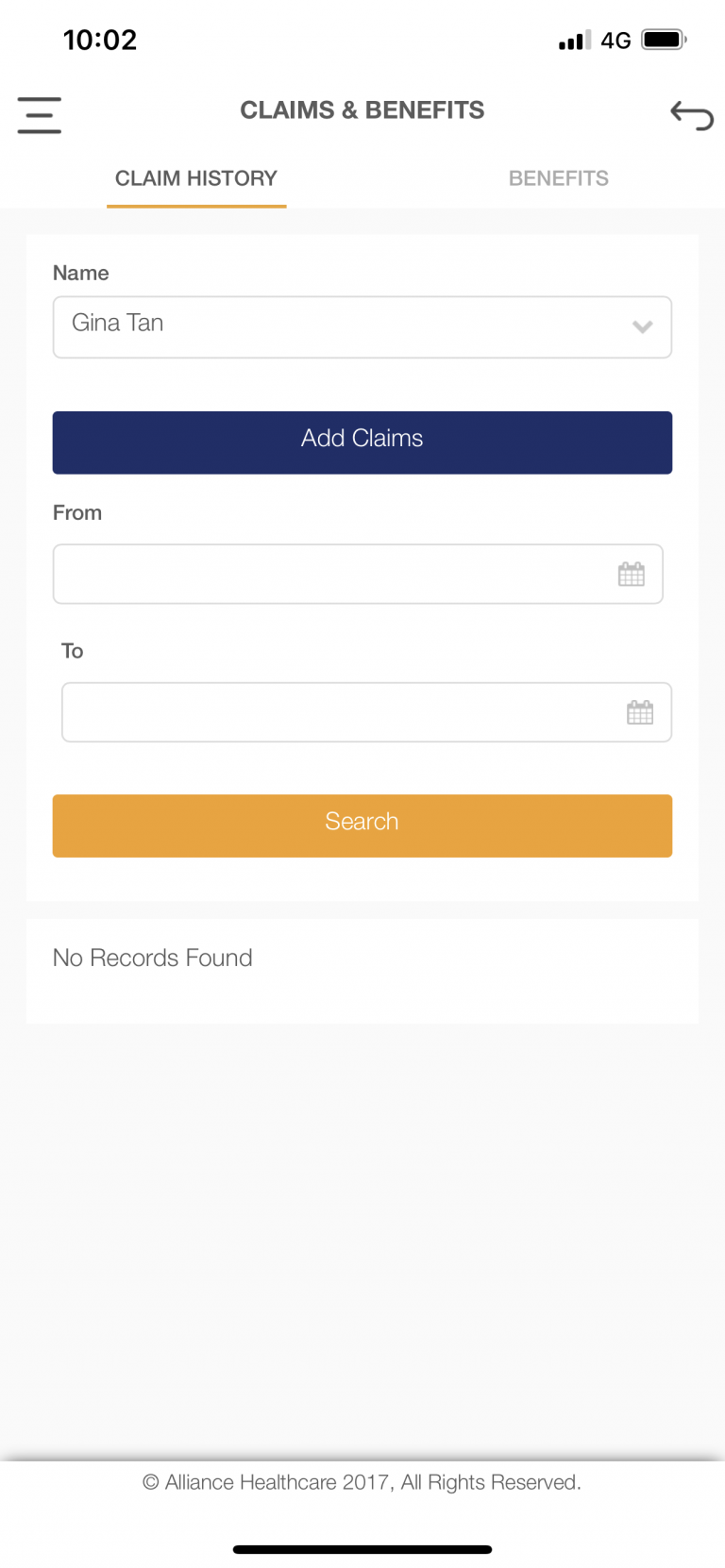The image displays a smartphone screen showcasing an application interface. At the top-left corner of the screen, there are two out of four bars indicating a mobile data signal strength and a "4G" label next to it, signifying the network type. Additionally, the battery icon shows full charge. Below the status bar, the interface features three horizontal lines representing the menu option.

The main section of the screen includes tabs labeled "Claims" and "Benefits," with "Claims History" highlighted in orange, indicating the current selection. The user's name, "Gina Tan," is displayed along with a dropdown menu for additional options. The interface provides a search function with a calendar date range, featuring fields like "Add Claims From Date" and "To Date." 

A message in the center reads, "No records found," signifying that there are no claim entries within the specified date range. At the bottom of the screen, there is a copyright notice: "Copyright Alliance Healthcare 2017, all rights reserved," followed by a black bar extending across the screen's width.